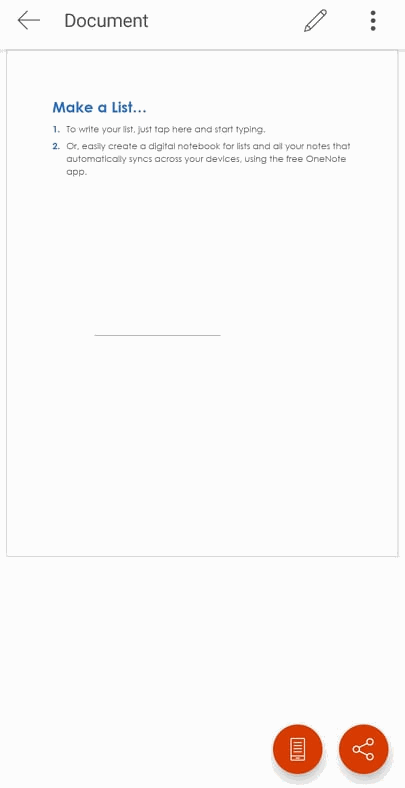The image showcases a minimalist mobile interface of the OneNote app. At the top of the screen, the word "Document" is prominently displayed, suggesting the opening of a new note. Below this, the text guides users to "Make a list," prompting them to tap a specific area to start typing. The app offers the functionality to create bulleted or numbered lists, allowing users to switch between these formats as needed.

At the bottom of the screen, two buttons are visible. One resembles a share button, indicating an option to share the note, likely represented by interconnected nodes and lines. The other button appears to be a phone icon, possibly offering a switch to the desktop version of the site or app.

The top section features several icons: an ellipsis for more options, a pencil for drawing or annotating with a finger, and a back button next to the word "document," hinting at the ability to navigate to different kinds of notes. The interface is presented in a clean, compact fashion typical of mobile applications.